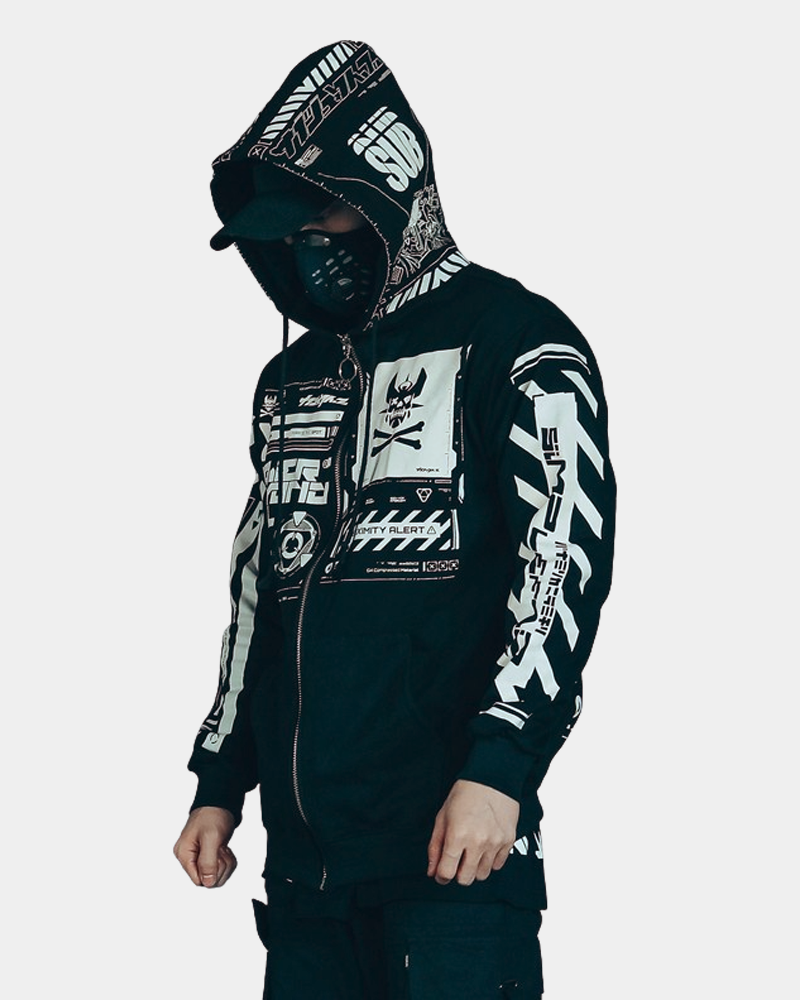The image features a Caucasian man modeling an outfit predominantly in shades of green and black. The ensemble includes green pants and a green hoodie adorned with white text and multiple sponsorship logos. Notably, the word "SUB" is prominently displayed in white on the hoodie. The man is also wearing a green baseball cap beneath his hood and a green mask covering much of his face. His body is positioned slanted toward the right, with his head angled downward. The model is facing slightly to the right, spanning from the middle bottom of the image to the top, set against a plain, pearl white background. He appears to be a performer, athlete, or skateboarder, indicated by the sporty nature of his attire and the various sponsor logos. The green strings typical of a hoodie hang down from its top. The overall scene suggests a promotional image for a clothing line, possibly associated with sports or streetwear.